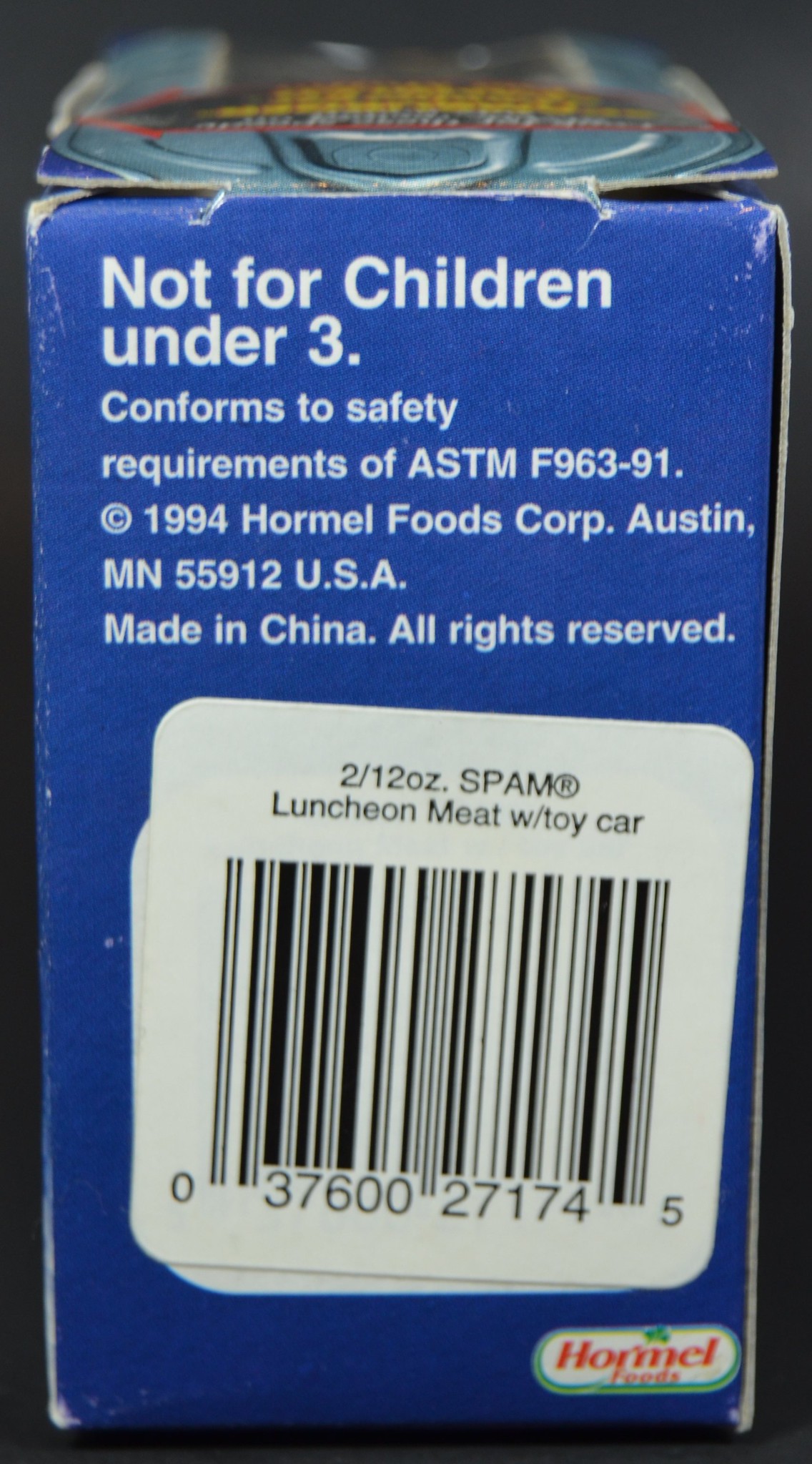The image features a close-up of a label on the side of a blue box of Spam luncheon meat, set against a black background. The top of the box has an image resembling the metal top of a Spam can, with silver detailing, yellow writing, and a red outline. Prominent white text on the side of the box warns: "Not for children under three," followed by "Conforms to safety requirements of ASTM F963-91." Below this, the label reads "Copyright 1994, Hormel Foods Corp, Austin, Minnesota 55912, USA, all rights reserved. Made in China." At the bottom part of the side label, there's a large barcode sticking out slightly angled to the right, accompanied by text indicating "Spam luncheon meat with toy car." The Hormel Foods logo is also visible in red letters against a white background at the bottom right of the box.